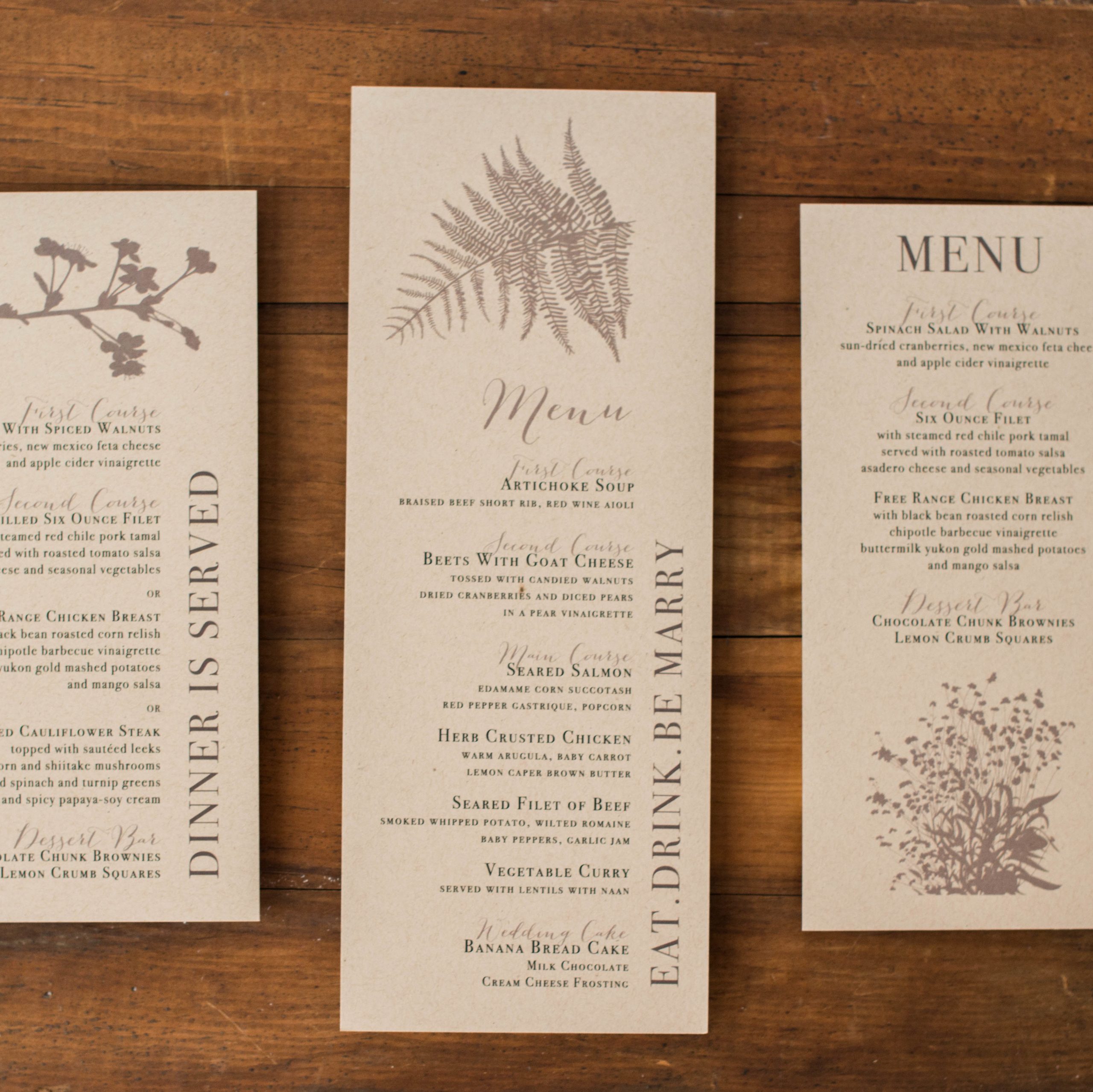The image features three pieces of sandy, tannish-brown stationery set against a dark wood surface, likely a table. Each piece of stationery is adorned with floral or plant-like designs, with the plant illustrations positioned differently on each: at the top for the left and middle pieces, and at the bottom for the right piece. 

Starting from the left, the first piece of stationery, titled "Dinner is Served" in sideways text, details a menu with a "First Course" featuring items such as spiced walnuts, New Mexico feta cheese, and apple cider vinegar. The "Second Course" includes dishes like a six-ounce filet, steamed red chili pork tamale with roasted tomato salsa, free-range chicken breast with black bean-roasted corn relish, chipotle barbecue vinaigrette, buttermilk Yukon gold mashed potatoes, and mango salsa. There is also the option of cauliflower steak topped with sautéed leeks and shiitake mushrooms, spinach and turnip greens, with spicy papaya soy cream. The "Dessert Bar" lists chocolate chunk brownies and lemon crumb squares.

The middle piece of stationery, containing the phrase "Eat, Drink, Be Merry" in a whimsical, period-separated format, also presents a multi-course menu. The "First Course" offers artichoke soup and braised beef short rib with red wine aioli. The "Second Course" features beets with goat cheese, candied walnuts, dried cranberries, diced pears, and pear vinaigrette. For the "Main Course," options include seared salmon with edamame corn succotash and red pepper gastrique, herb-crusted chicken with warm arugula, baby carrots, and lemon caper brown butter, seared filet of beef with smoked whipped potatoes, wilted romaine, and garlic jam baby peppers, as well as vegetable curry served with lentils and naan. The dessert is a wedding cake made of banana bread with milk chocolate cream cheese frosting.

The rightmost piece of stationery, simply headed "Menu," reiterates some of these offerings. The "First Course" includes a spinach salad with walnuts, sun-dried cranberries, New Mexico feta cheese, and apple cider vinaigrette. The "Second Course" mirrors an earlier menu with a six-ounce filet and steamed red chili pork tamale served with roasted tomato salsa and seasonal vegetables, as well as free-range chicken breast options with black bean-roasted corn relish, chipotle barbecue vinaigrette, and buttermilk Yukon gold mashed potatoes. The “Dessert Bar” again features chocolate chunk brownies and lemon crumb squares.

Taken together, these three pieces of stationery likely serve as the wedding menu, offering a variety of culinary delights set against a rustic, elegant wooden backdrop.